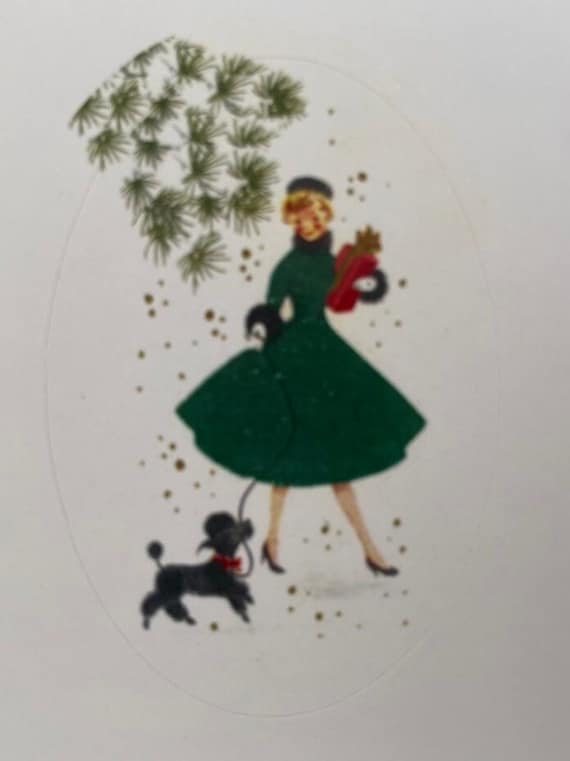In this blurry cartoon image, we see a lady dressed in a green 1950s-style dress with black-trimmed sleeves. She has yellow hair adorned with a hat and blushes on her cheeks, giving her a classic, nostalgic appearance reminiscent of Donna Reed or Patty Duke. The lady is holding a red-wrapped gift in one hand and a leash in the other, attached to a trimmed black poodle sporting a red collar. The poodle exudes an air of arrogance, prancing around happily. The scene includes subtle details like leaves in the top left corner and a gray, bleak background, which contributes to the intentionally blurry quality of the artwork. Despite the poor picture quality, the cute attitude of the little dog stands out vividly.